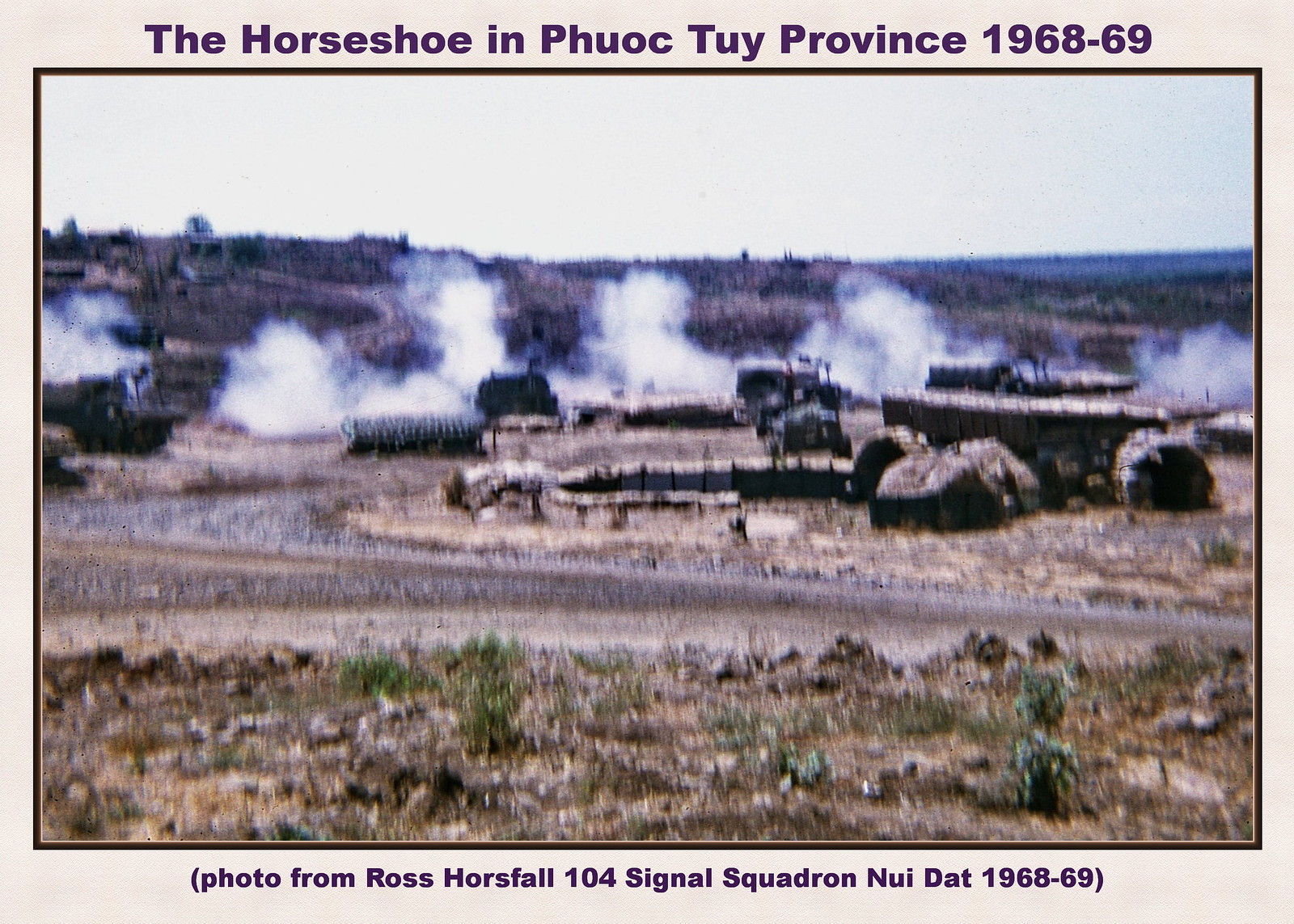The photograph captures a scene from what appears to be a military camp in Vietnam, specifically in the Horseshoe area of Phuoc Tuy province during 1968-69. In the foreground, there is some short green grass and brownish bushes. Following that, there is a gravel road with scattered vegetation and a few trees. Numerous billows of white smoke rise across the image, suggesting the presence of trains. In the midground, there are makeshift straw huts, barrels, and military equipment, including trucks. Off to the left, an army truck is especially discernible. The landscape is predominantly dry, with sparse grassy areas and dirt patches. In the background, distant hills and barren mountains can be seen under a white sky. The purple text at the top of the photo reads "The Horseshoe in Phuoc Tuy province, 1968-69," while at the bottom, similar text mentions "photo from Ross Horsefall, 104 Signal Squadron, Nui Dat, 1968-69." The overall image has a dated appearance, indicative of its historical context.